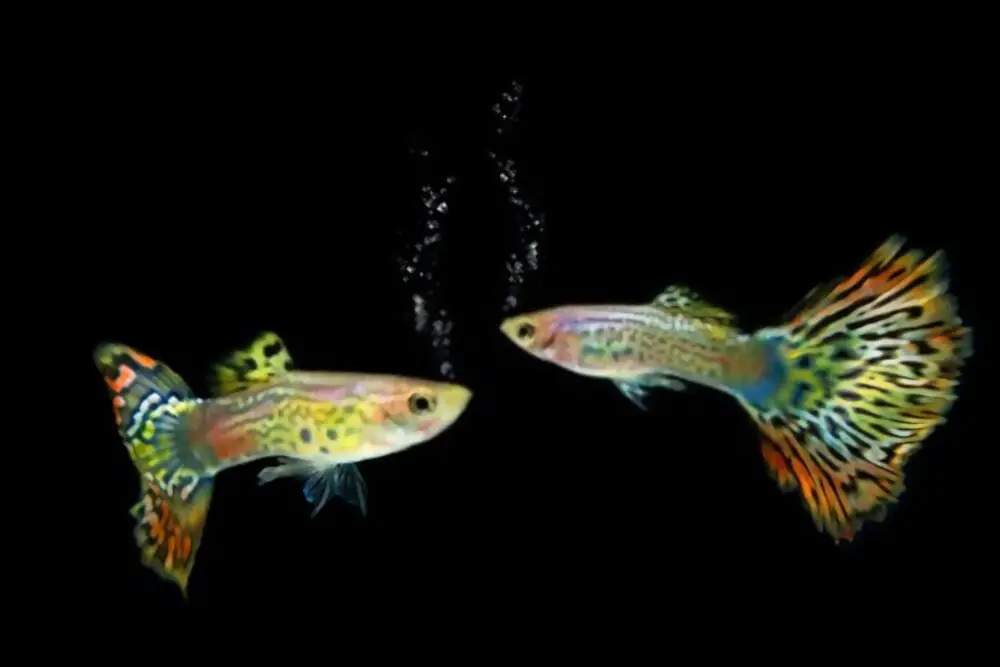In this striking image, two opalescent fish are showcased against a completely black background. The fish, which appear to be facing each other, are vividly multicolored and adorned with intricate patterns. The fish on the left is slightly larger and is positioned slightly lower than the one on the right, which is more slender and higher up in the frame. These fish have remarkable tails that are feathery and brush-like, with vibrant colors including orange, white, and yellow, accented by black speckles that resemble a monarch butterfly's wings.

Their bodies are predominantly yellow and pink with tinges of blue and a muted speckle design that varies in size and depth, akin to the spots on a wildcat. The larger fish on the left displays a more expansive dorsal fin adorned with yellow and black spots, while the right fish’s fin is taller and more prominently yellow. The entire scene, accentuated by the stream of bubbles rising from each fish’s mouth, presents a beautiful and almost otherworldly tableau of these two magnificent creatures meeting in the dark waters.